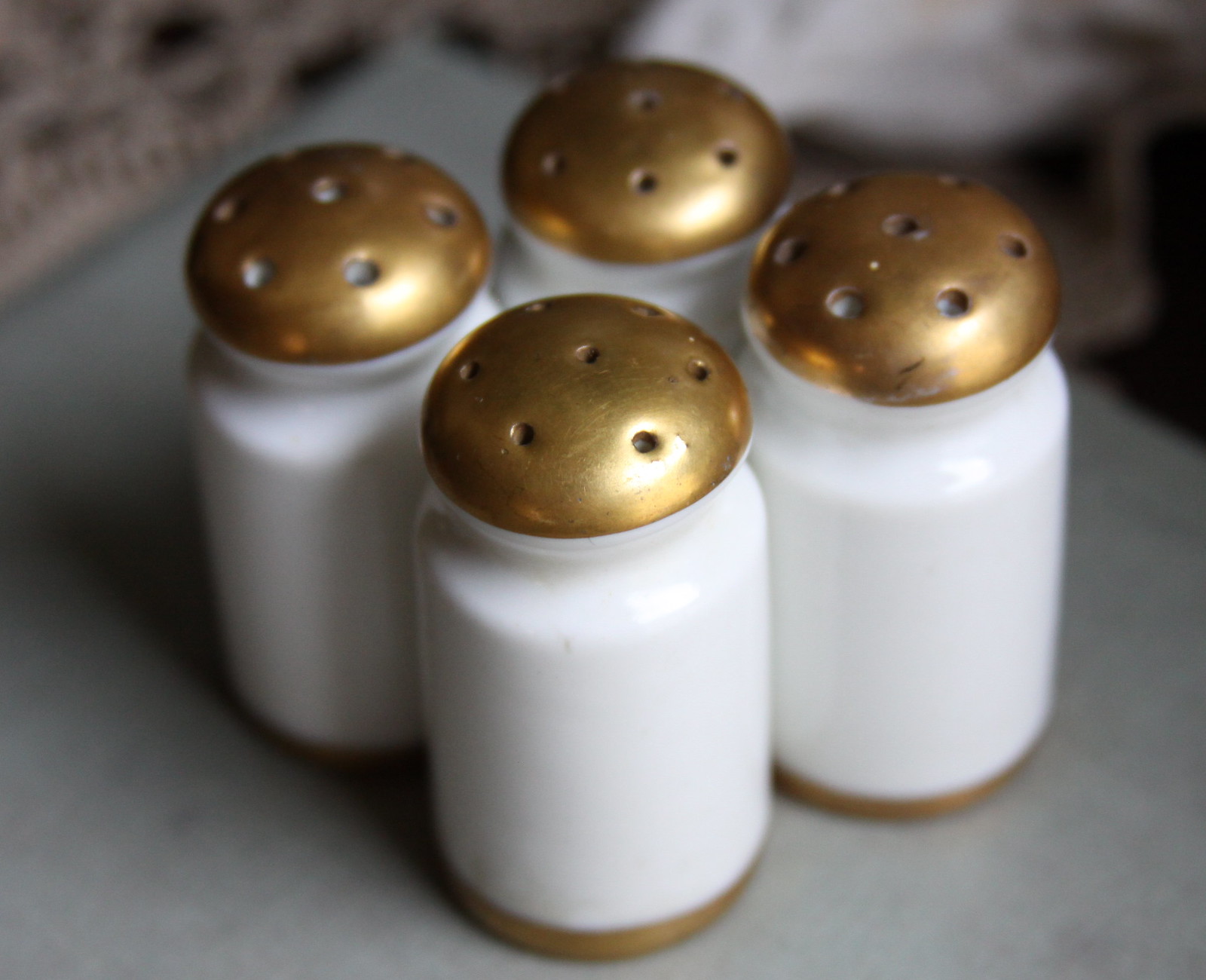The image showcases a neatly arranged collection of four cylindrical salt or pepper shakers, each with a distinct, vaguely mushroom-like appearance. They are primarily composed of glossy white ceramic with a polished metallic finish in a gold or possibly copper tone on both the caps and bottoms. Each shaker features a notch just below the cap, giving it a unique segmented design. The caps are adorned with seven holes: one centered hole surrounded by six others, arranged in a diamond formation with two smaller and four larger holes.

The shakers are placed in a square formation atop a whitish or gray tray, which is itself set against a slightly blurred backdrop. The background includes a pink knit doily in the upper left corner and a piece of paper in the upper right, though these elements are less distinct. The wooden texture of the underlying table adds a warm, rustic touch to the scene. Some of the caps appear weathered or patinaed, hinting at frequent use, and small traces of leftover salt are visible, confirming their use as salt shakers.